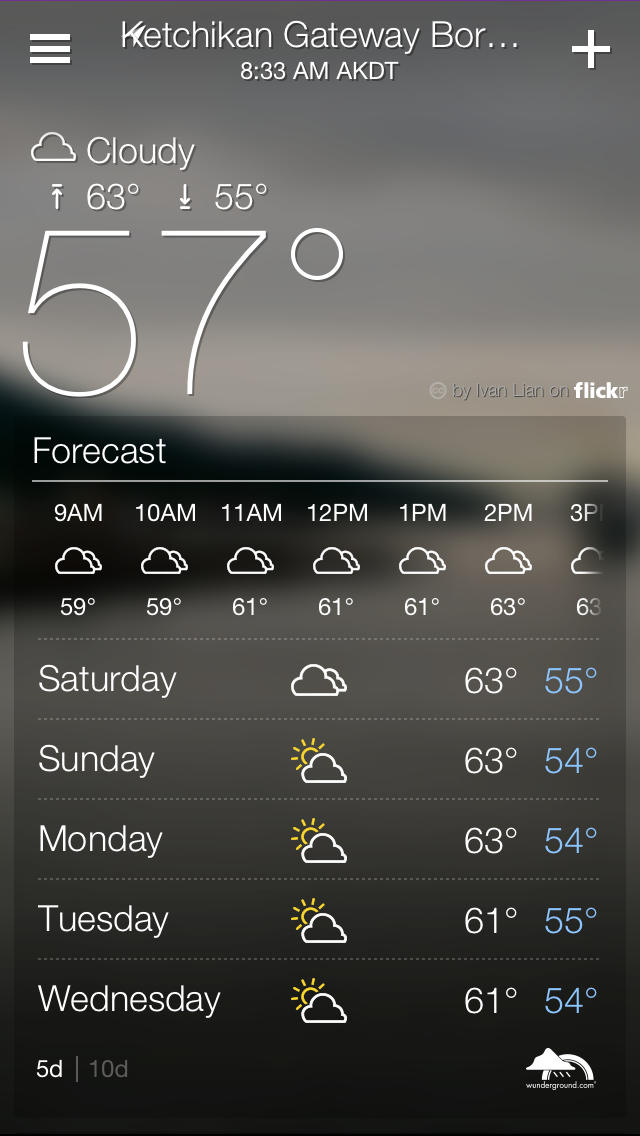The screenshot, taken at 8:33 a.m. AKDT, displays the weather forecast for Ketchikan Gateway, as shown in a weather app. The five-day option is selected from the available 5-day and 10-day forecast options. The current weather in Ketchikan is cloudy with a temperature of 57°F. For today, the expected high is 63°F and the low is 55°F, indicating minimal temperature variation. The upcoming week features consistently cloudy weather with temperatures remaining remarkably steady. The next three days forecast highs of 63°F, followed by slightly cooler highs of 61°F later in the week. Lows throughout the week hover around 54°F to 55°F, with a slight hint of sunshine towards the weekend. The constant weather reflects a stable and mild climatic condition in the region.